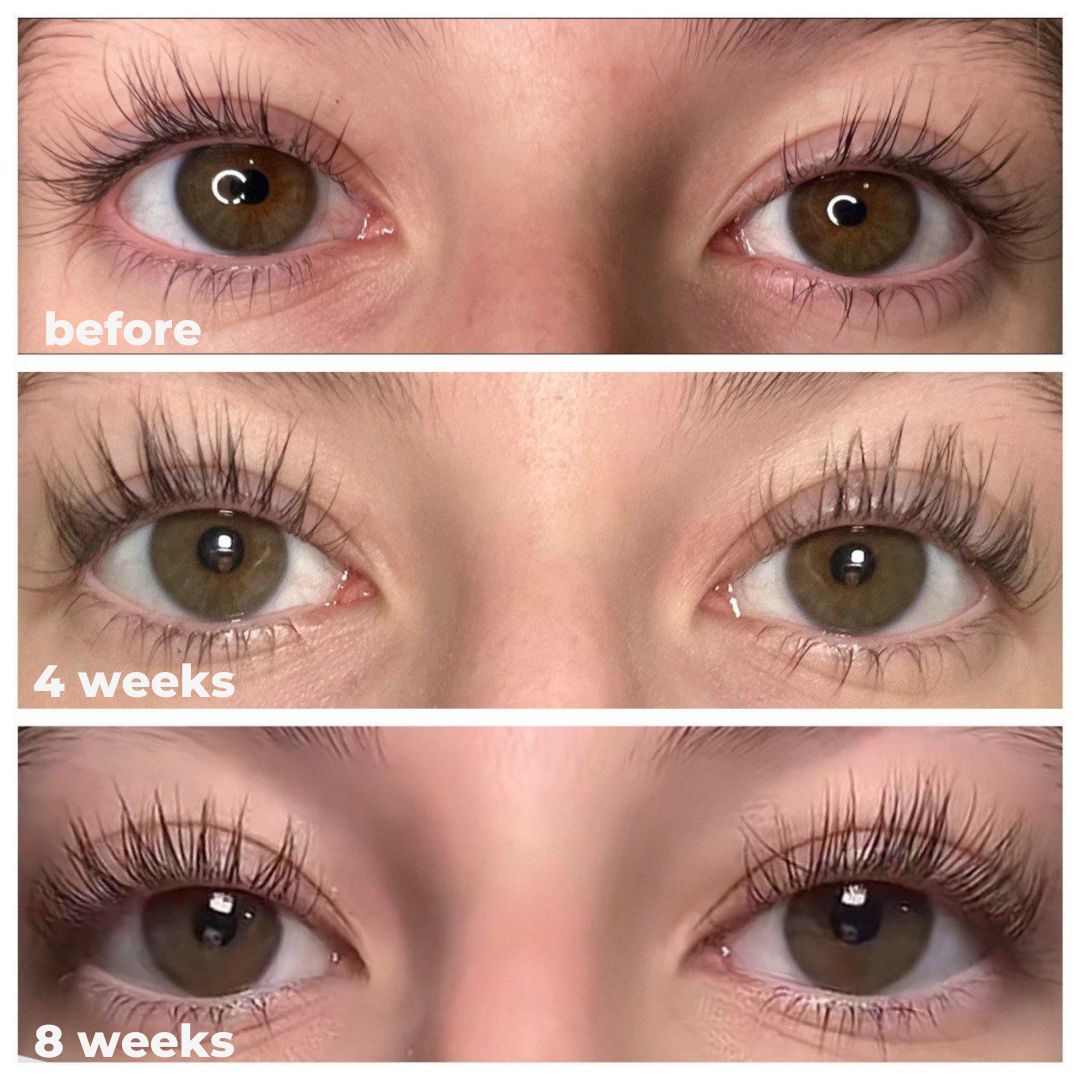The photograph showcases a sequence of three close-up images of a young woman’s eyes, likely of European descent, with fair skin and hazel eyes. Each rectangular image is aligned vertically, marked by text denoting time progression: "Before" at the top, "Four Weeks" in the middle, and "Eight Weeks" at the bottom. In the "Before" image, her eyelashes appear sparse and wispy. Progressing to the "Four Weeks" image, there is a noticeable increase in the fullness and thickness of her lashes. The "Eight Weeks" image displays a significant transformation with markedly thicker, longer, and more filled-in eyelashes. Bright lighting highlights the details in her irises and the dramatic change in lash density over time.